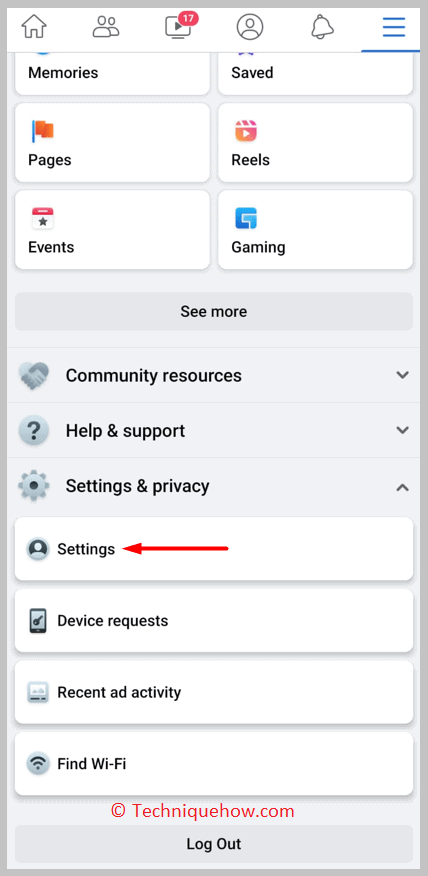This image is a screenshot showing a detailed section of a user interface, likely from a social media platform or a similar application. The entire perimeter of the screenshot is bordered by a thin gray line. The background of the interface is predominantly white.

At the top, there is a navigation bar with several icons: a home icon, a figure of two people, and a square with a right-pointing triangle inside it. Above the square icon, there is a small red circle with the number '17' displayed inside it, suggesting unread notifications. Continuing to the right, there is a round icon with a person's silhouette, a bell icon, and three horizontal blue lines stacked on top of one another.

Beneath the navigation bar, there are several labeled panels. On the left side, the panels are titled "Memories," "Pages," and "Events." On the right side, the top panel is labeled "Saved," followed by "Reels" and then "Gaming."

In the center of the interface, there is a gray banner, which features a darker and lighter gray gradient, displaying the text "See More." 

Below this banner, there is a dropdown menu with several options: "Community Resources," "Help and Support," and "Settings and Privacy." 

Further down, four white-background panels are listed with headings and sub-sections. These include "Settings" with a red arrow pointing towards it, "Device Requests," "Recent Ad Activity," and "Find Wi-Fi." At the bottom, there is red text that says "Copyright Technique How Calm," and beneath it in black print, the word "Log Out" is displayed.

The detailed elements of this interface provide a thorough overview of user interaction options and available features within this application.